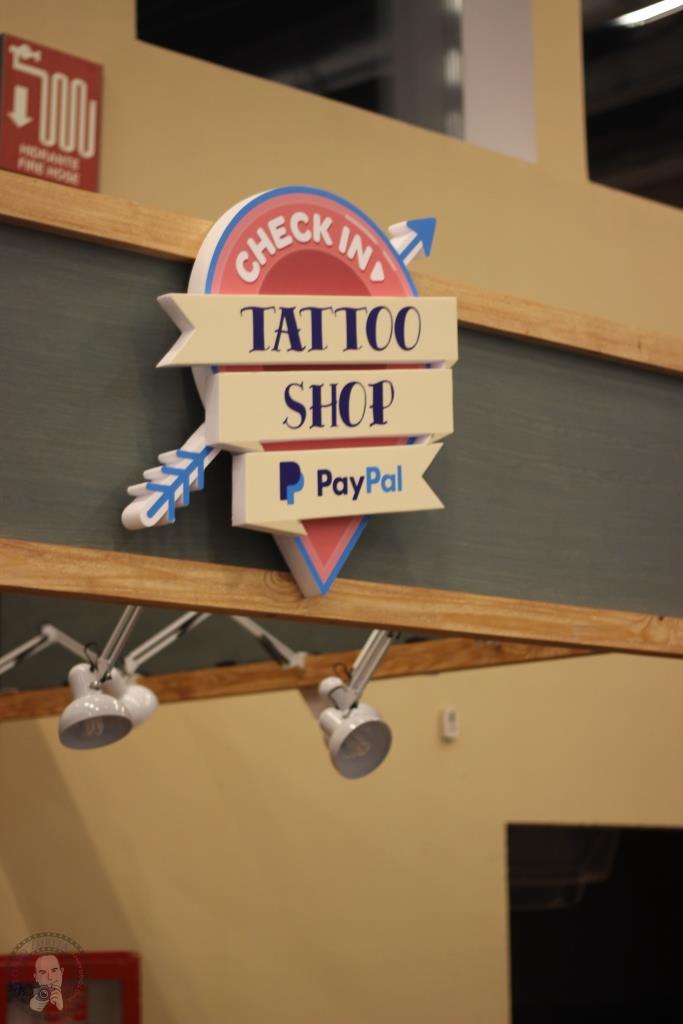The vertical rectangular photograph depicts the facade of a multi-story concrete building with wood trim. A person stands in front of a lower window. Above this window, there is a prominent sign for a tattoo shop. The sign is a large red circle with a blue arrow running from the lower left to the upper right, featuring white text that reads "Check-in" and pointing towards a specific entrance. Included within the sign, in separate blocks, the words "Tattoo Shop" and "PayPal" are also displayed. The vibrant PayPal logo stands out vividly against the weathered colors of the sign. Mounted on the wooden board above, the sign is illuminated by movable, metal lights with white shades, directing light downwards. Skylights and an emergency exit indicator can be seen above, hinting at the building's utilitarian design.